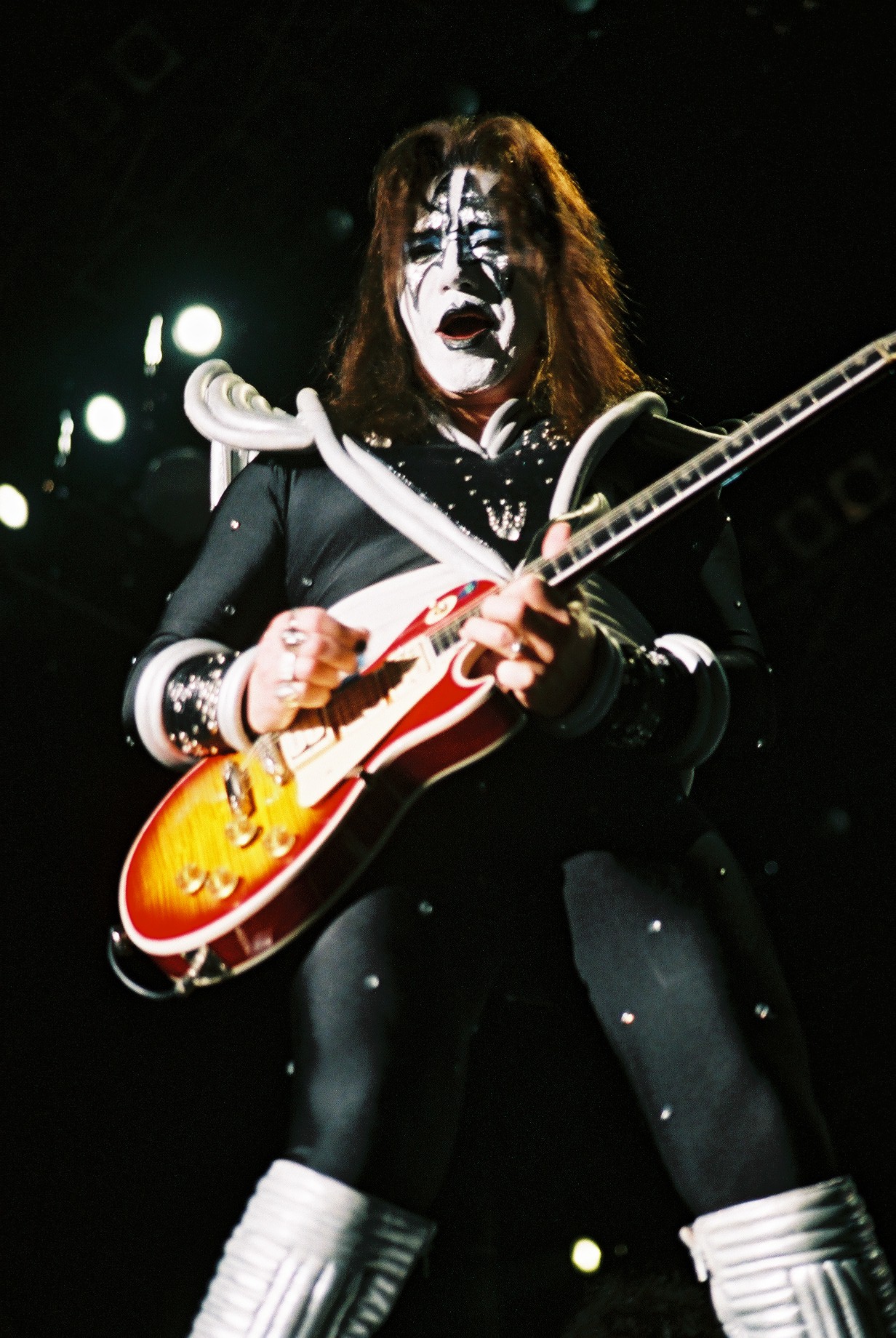The photograph captures a man, resembling a member of the rock band KISS, performing on stage. His face is elaborately painted with white makeup, featuring intricate black designs and blue accents around the eyes, giving him a striking appearance. He has long brown hair that cascades over his shoulders. His outfit is predominantly black, adorned with black gemstones and white sequined dots. He wears a textured accessory, possibly a collar with rhinestones and a white border, enhancing the ornate look. His attire includes a black tight shirt and black leggings, paired with distinctive white boots. He holds an electric guitar that is yellow at the base, with red accents and a white trim, and it features a white strap. The stage is dimly lit, with a series of stage lights above and one positioned beneath his spread legs, intensifying the dramatic atmosphere of the performance. The camera angle from below amplifies his commanding presence on stage.